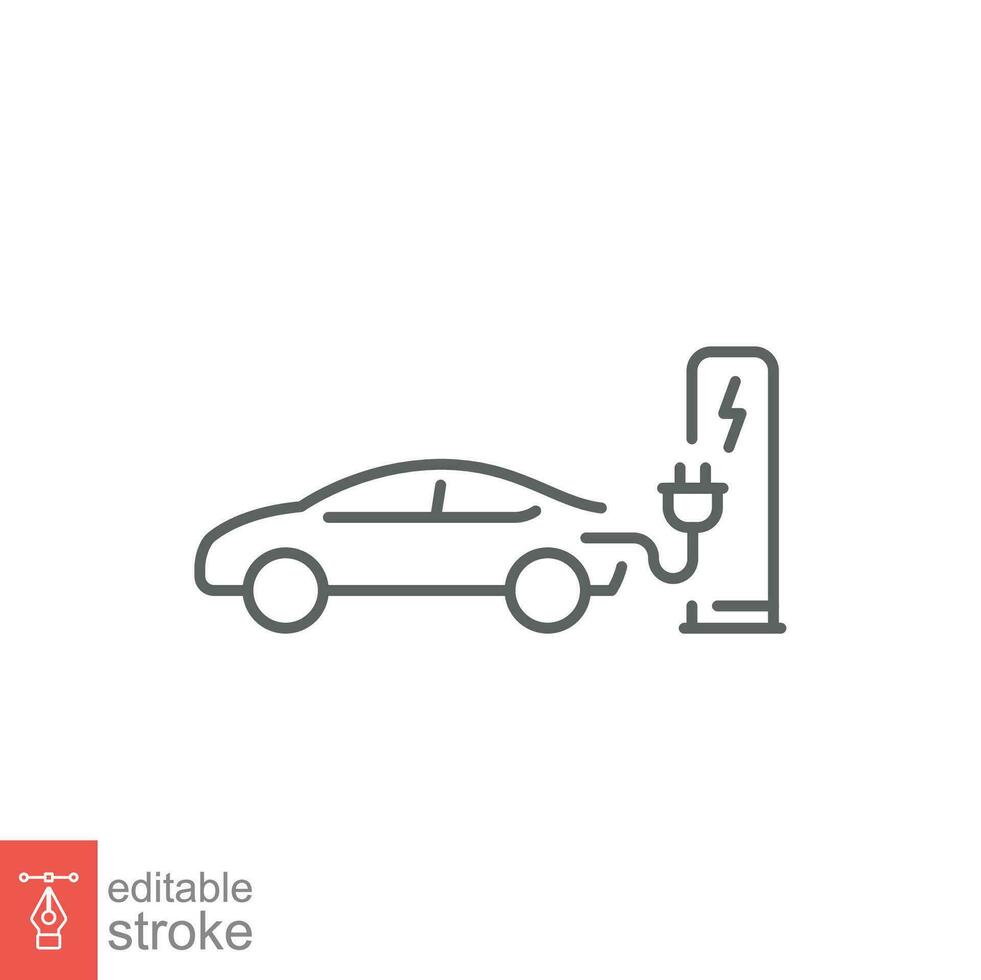The image features a black-and-white vector graphic that serves as a logo for an electric car charging station. The illustration shows a stylized car with an electrical cord extending from its rear, with the prongs of the plug curving upward. The design is minimalist with open outlines, meaning the lines defining the car, windows, and charging station do not connect fully—leaving deliberate gaps. Adjacent to the car, a rounded rectangle with a lightning bolt symbol represents the charging station. In the bottom left corner, there's an orange-and-gray logo depicting a pen tip with three nodes, accompanied by the text "EDiTABLE Stroke."